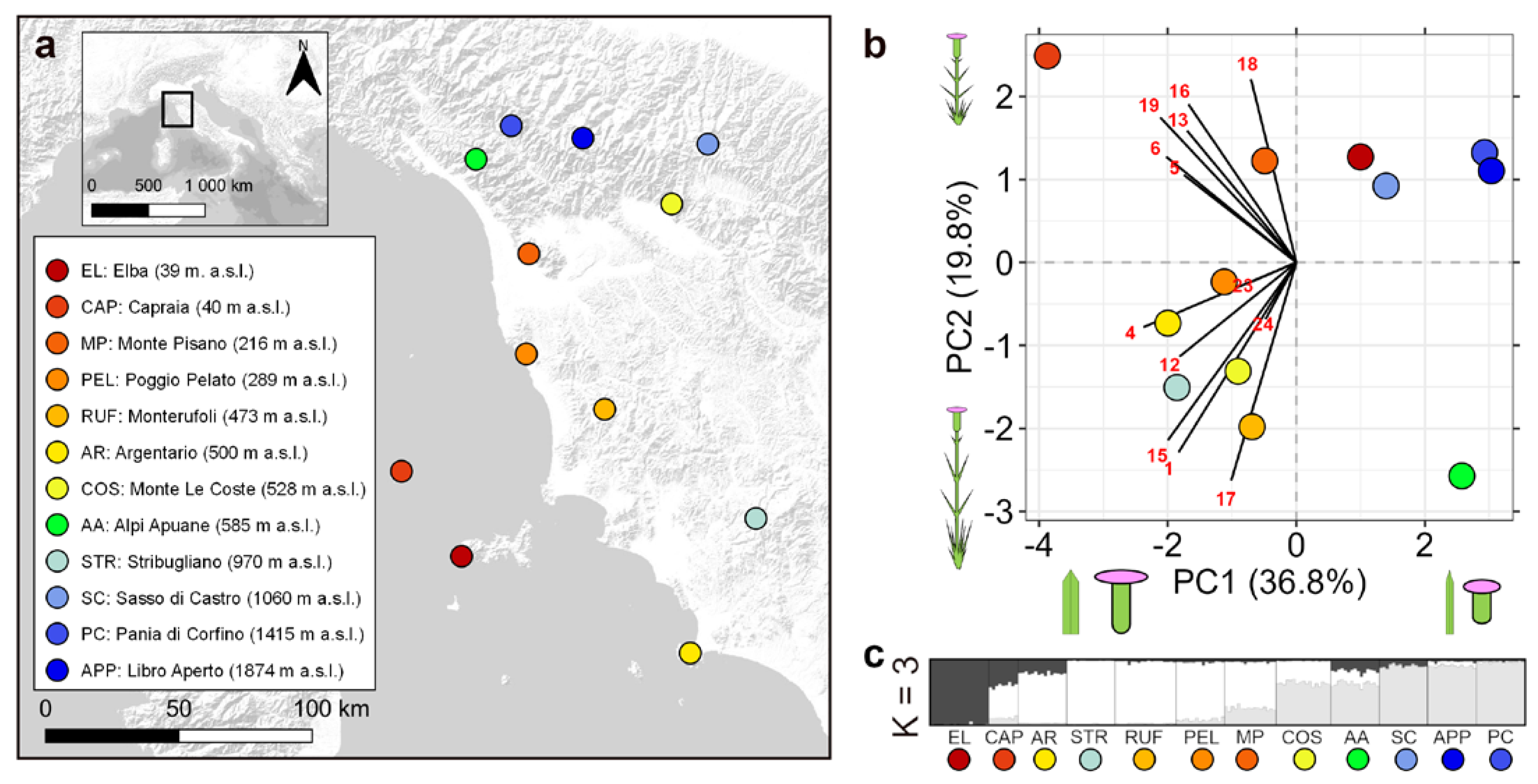The image features two main sections organized in a landscape orientation, divided into two halves. The left side presents a black-and-white map, likely of a coastal region, adorned with a variety of colored dots—green, blue, light blue, yellow, orange, teal, and red—each representing different locations. The legend accompanying the map identifies labeled points such as AR for Argentario (yellow dot) and APP, Libro, Umberto (dark blue dot), amidst numerous other locations like Elba, Capra, Monty, and La Costa.

The right side contains a multi-quadrant graph described as a coordinate system extending from minus 4 to 2 on the x-axis and minus 3 to 2 on the y-axis. This graph highlights dots scattered across the quadrants and includes labels like PC2 (19.8%) and PC1 (36.8%) on the sides. Additionally, lines radiate from the center towards the left, adorned with various numerical indicators. Below this graph lies another, more intricate line graph. This lower graph, noted with K=3, also incorporates the color-coded dots, aligning them with their respective labels and displaying peaks in a horizontal bar layout.